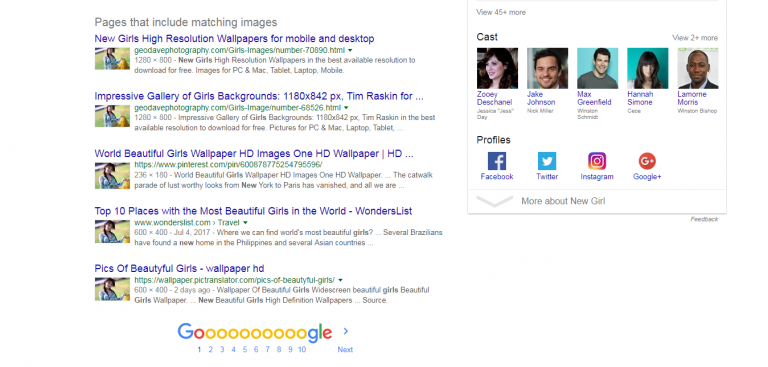"Explore the Top 10 Destinations Known for their Breathtakingly Beautiful Women: A Collection of Stunning Wallpaper-worthy Images Featuring the World's Most Gorgeous Girls. This gallery also highlights captivating snapshots of the cast from the beloved series 'New Girl,' including Zooey Deschanel, Jake Johnson, Max Greenfield, Hannah Simone, and Lamorne Morris, offering a delightful blend of beauty and celebrity charm."